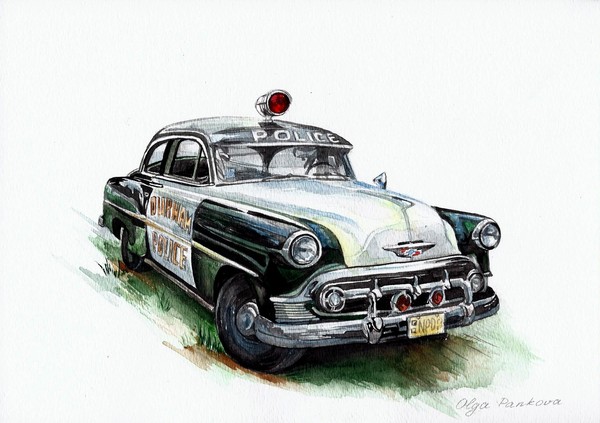This detailed illustration depicts a vintage 1950s police car rendered in black and white. The vehicle has a distinctive thick silver bumper adorned with yellow blinker lights on each side and features a barely visible car emblem on its hood. Prominently displayed on the left side, across the passenger door, is the text "Durham Police," suggesting a link to Durham, possibly in North Carolina or South Carolina. The car's design includes dual headlights flanking the front hood. On the car's roof sits an iconic, single red police siren light. The drawing, which also captures the texture of grass and mud beneath the car, appears to be done in watercolor. Notably, the artist's signature, "Olga Pankova," is visible in the bottom right corner of the artwork.